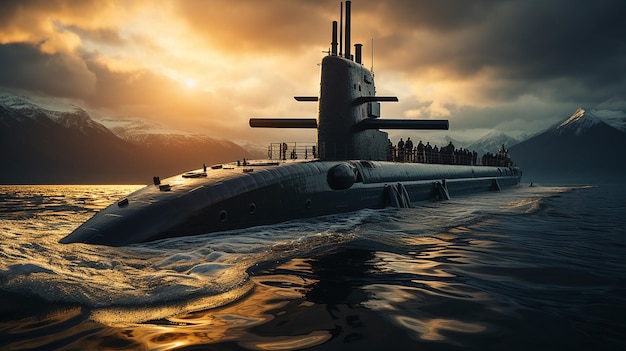The image is a striking, AI-generated graphic that boasts realistic comic book-level detail. It depicts a powerful and evocative scene of a military submarine breaking the surface of dark, tumultuous waters. White foam splashes up on either side of the long, oval-shaped vessel with its prominent central tower. The submarine's top features multiple protruding pipes and rods, and there's a black railing encircling the upper deck to prevent the numerous servicemen, visible as shadowy outlines, from falling off. Surrounding this dramatic focal point are towering mountains: some on the left, large and foreboding, stretch towards the center, while more distant peaks on the right are pointed and snow-capped. The sky above is a dynamic mix of conditions, predominantly dark, stormy, and cloud-filled, with patches of orangish hue from the setting or rising Sun breaking through. This detailed scene captures a compelling moment, blending elements of nature's fury with military precision.